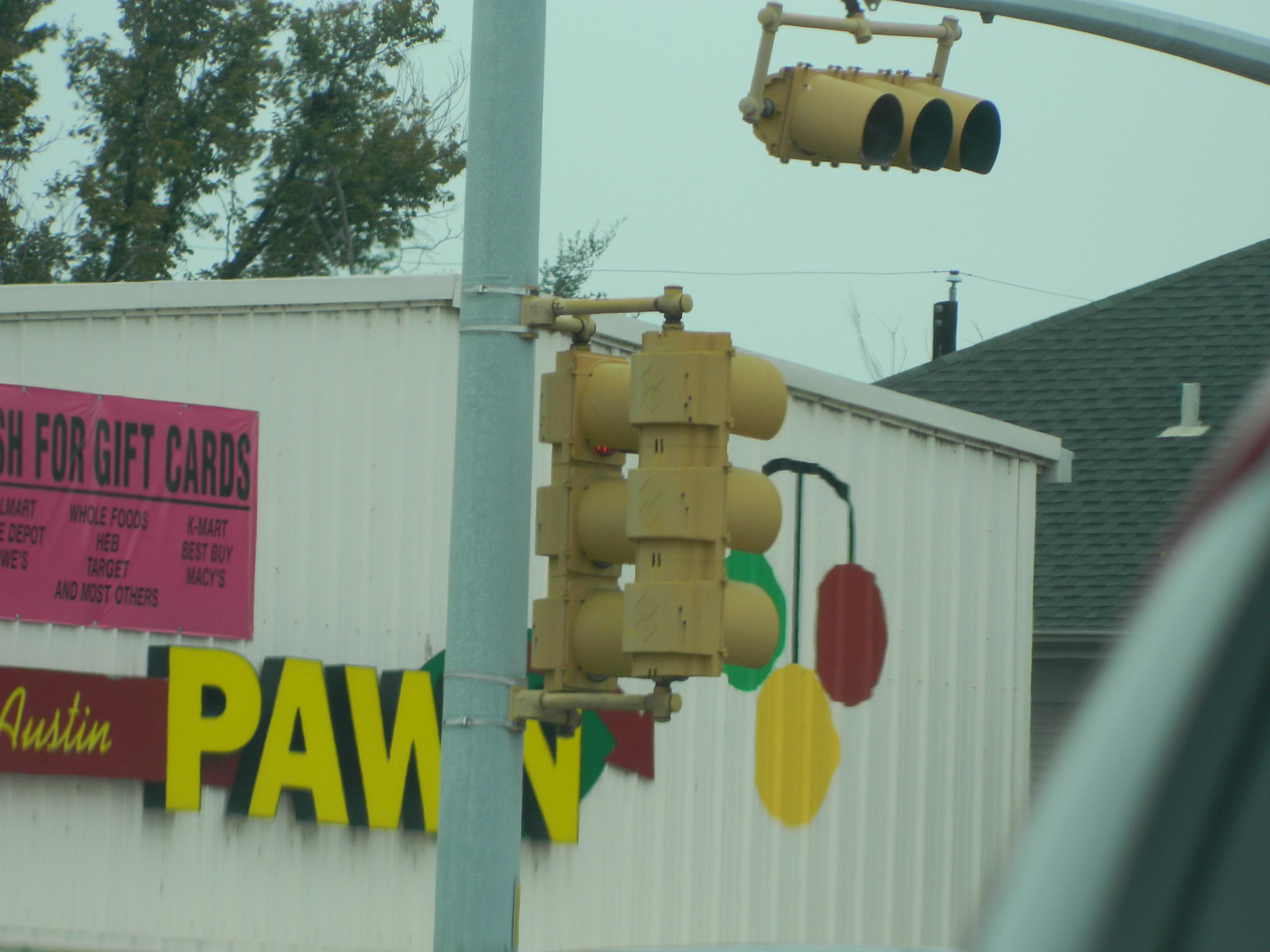The image depicts an overcast or pre-rainstorm sky, casting a hazy, dark aura over the scene. At the heart of the photo is a metal pole supporting two vertically oriented traffic lights and a third set of traffic lights mounted horizontally atop the image. None of the lights are facing the viewer, indicating an intersection from a different angle. 

In the background, a white, generic metal building presumably houses a pawn shop, as suggested by the partially visible large yellow "PAWN" lettering on the building. Alongside "PAWN," there is a maroon rectangle reading "Austin" in yellow letters. Adjacent to this sign, a design features green, maroon, and yellow orbs, likely a store logo.

Additionally, the building sports a pink banner with the visible words "for gift cards" in black letters, hinting at a phrase such as "cash for gift cards." Over to the right side of the image, a tree's branches extend above the building, and the top of a shingled roof with a small vent from another structure can be seen, accompanied by some background power lines. The overall scene suggests a quiet moment at an intersection framed by commercial and residential elements.